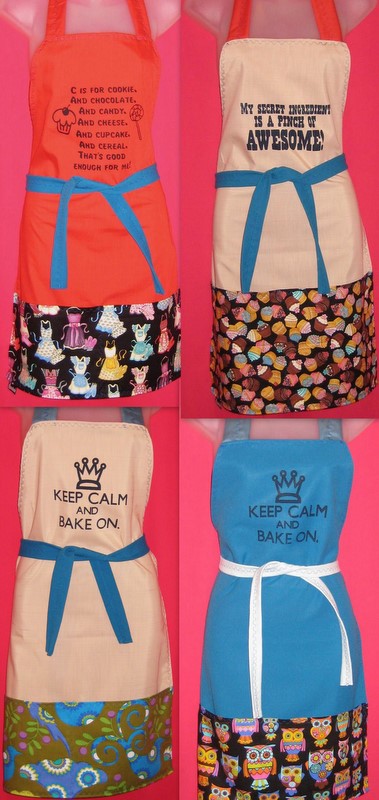This composite image features four different baker's aprons, each displayed over skirts with unique patterns against pink backgrounds in varying shades. In the upper left-hand corner, a coral-colored apron with a turquoise tie showcases a line drawing of a cupcake and a lollipop, accompanied by the whimsical text, "C is for cookie and chocolate and candy and cheese and cupcake and cereal. That's good enough for me." Below this apron, the mannequin dons a black patterned skirt. The upper right apron is tan with a blue tie, emblazoned with the phrase, "My secret ingredient is a pinch of awesome," over a cupcake-patterned skirt. In the lower section, two aprons share the slogan "Keep calm and bake on" accompanied by a small crown graphic. The left apron is tan with a matching blue sash, and the right apron is blue with a white sash, with the corresponding mannequins wearing skirts featuring owls and other decorative designs. This visually appealing collection aligns to form a vertical rectangle, presenting an orderly yet charming display of distinctive aprons perfect for baking enthusiasts.